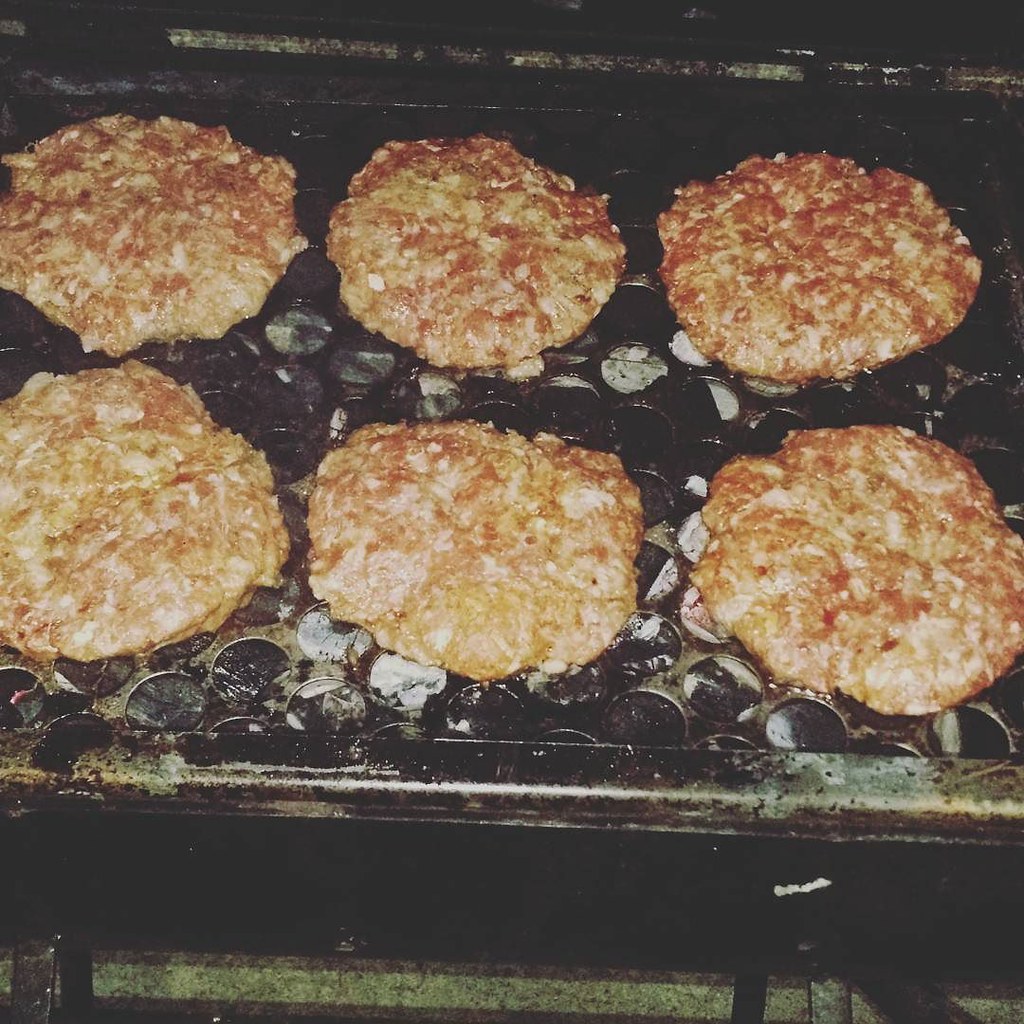This is a color photograph in a square orientation, taken from a 45-degree first-person angle looking down at a cooking surface. The image shows six food items, likely cheese and tomato pizzas, arranged neatly in two rows of three. Each pizza is irregularly shaped and fully covered with cheese and tomato, lacking the traditional exposed crust. They are placed on a metal grid that features a geometric pattern of circular holes and is set over what appears to be a charcoal base. The charcoal beneath includes chunks of both white and black pieces. Despite the presence of charcoal, there is no visible smoke or flames. The grill looks like a large, commercial-grade appliance that shows significant wear and tear, with dirty and greasy sections indicating heavy use. The background of the photo is dark and the quality hints that it might be an older image.